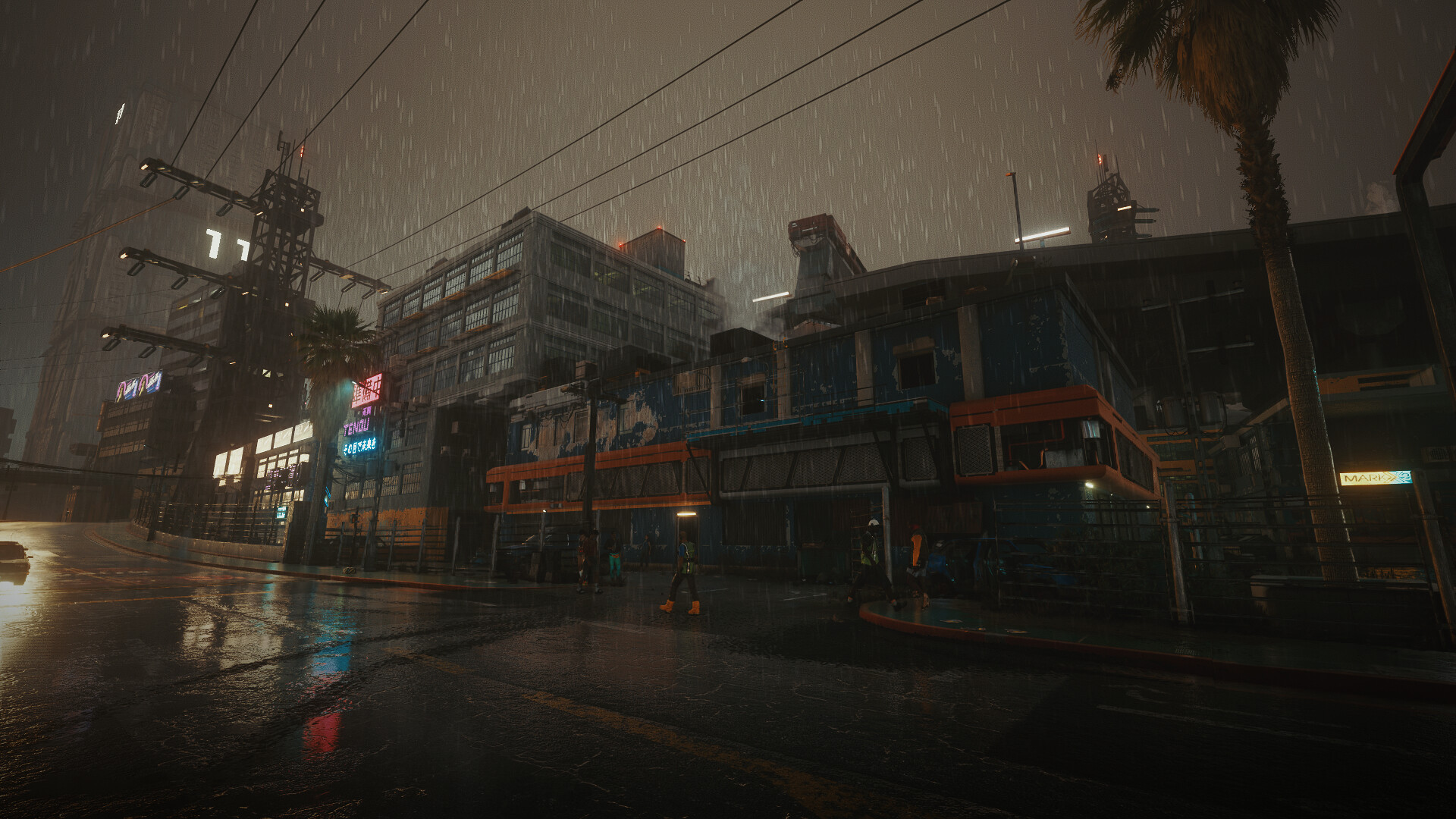In the image, a dense urban scene unfolds under a gray, rain-soaked sky. Persistent raindrops cascade from above, contributing to the reflective sheen on the wet street below. Overhead, utility poles strung with intricate webs of electrical lines stretch across the frame. The cityscape below is vibrant with life despite the dreary weather; neon signs in hues of blue, purple, and red illuminate storefronts and cast a colorful glow onto the pavement.

Shops with light emanating from their yellow-tinged windows add a warm contrast to the otherwise cool and muted atmosphere. These reflections dance subtly on the slick surface of the street, enhancing the visual depth of the scene. The architecture is modest, comprised of concrete and stone buildings, none towering too high, allowing for a more intimate urban experience. To the right, a street sign makes its presence known, while a lone palm tree stands amidst the rain, adding a touch of natural life to the otherwise concrete jungle.